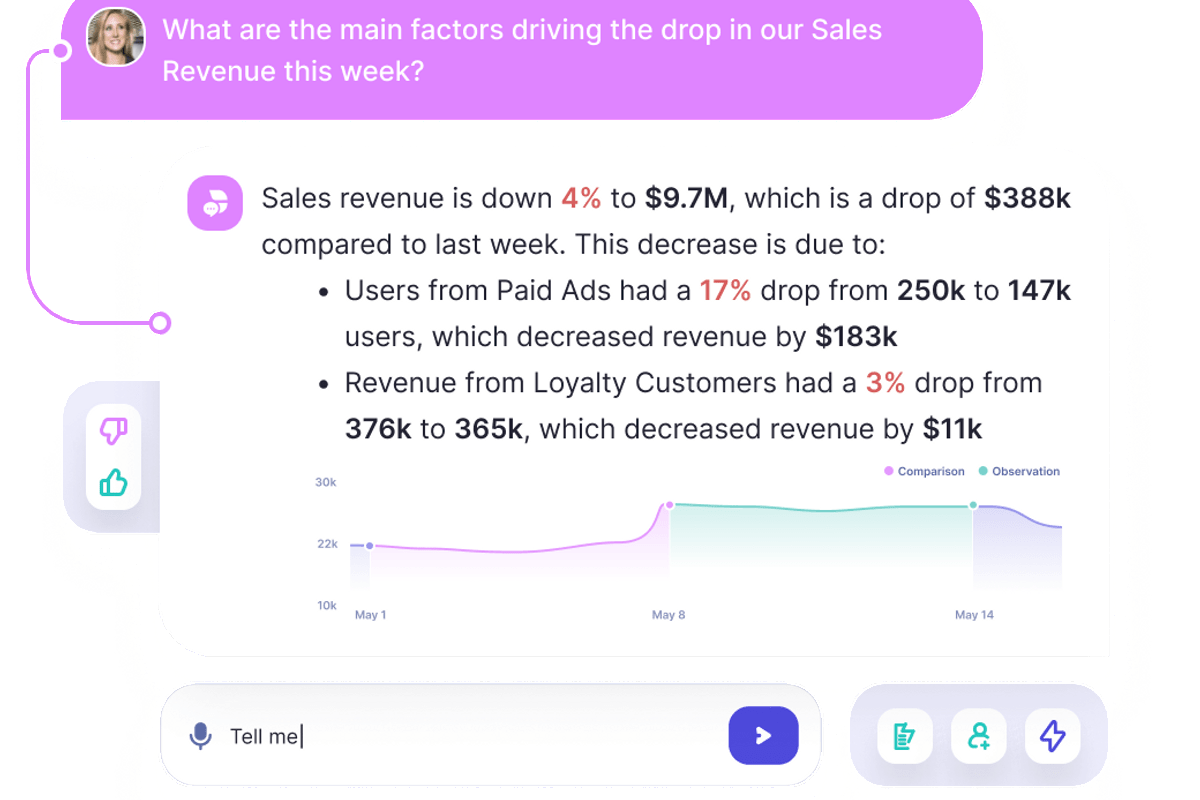In this detailed image, the top left corner features a circular profile picture of a woman. Adjacent to this profile picture, towards the right, is the text "What are the main factors driving the drop in our sales revenue this week?" The entire text area is set against a pink background. On the far left of this pink background, there's a purple line extending vertically down into another circle, intersecting at the middle left.

In the bottom left corner, there are pink thumbs-down and thumbs-up icons, positioned within a small white rectangle set against a larger gray rectangle. Notably, the thumbs-down icon appears above the thumbs-up icon. Moving to the right, in the bottom middle section of the image, the text "Tell me" is displayed alongside a small microphone icon.

Situated in the bottom right corner is a right-pointing arrow encased in a blue square border. Above this segment, a detailed graph is plotted. The graph charts a vertical range from 10K to 30K and spans horizontally from May 1st to May 14th.